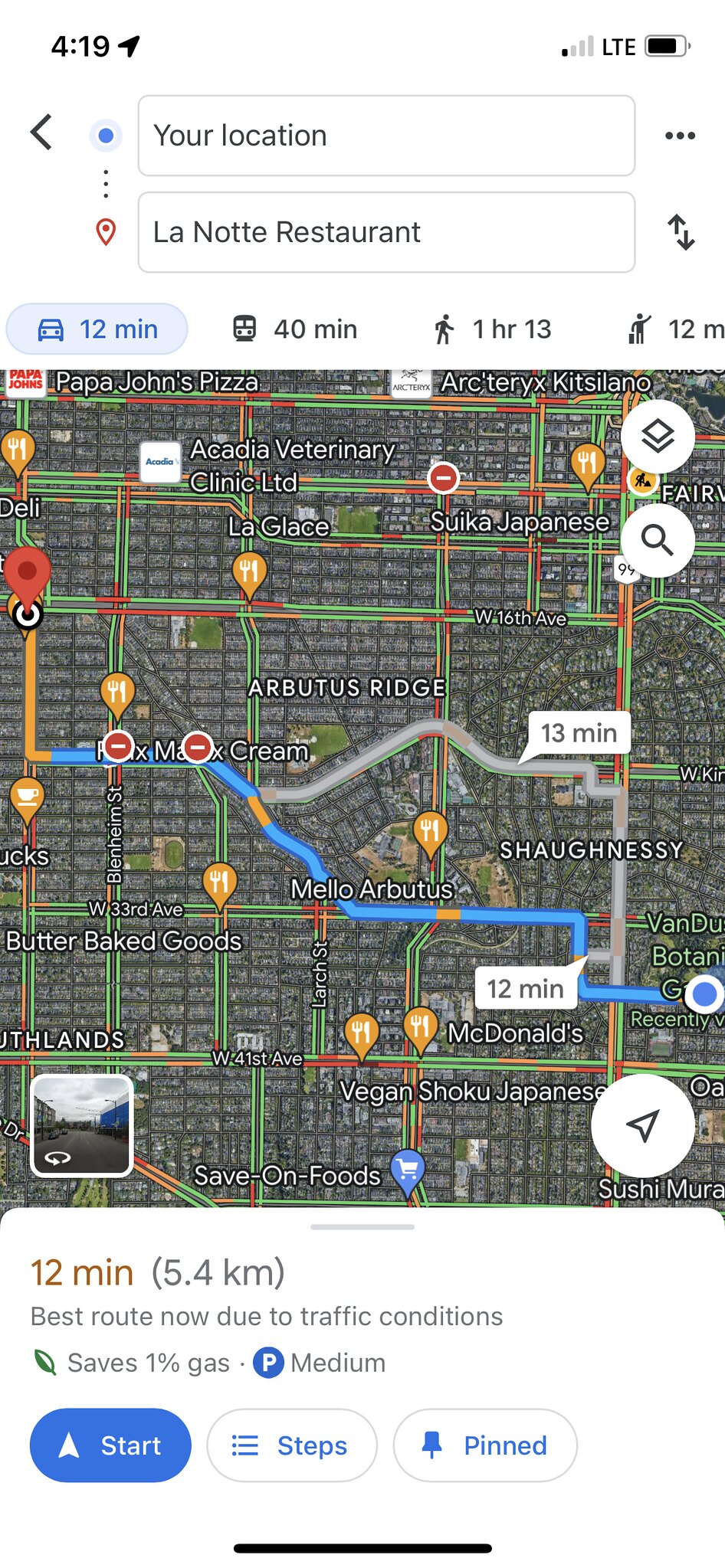This screenshot, captured on a smartphone at 4:19 PM, features a detailed view of a Google Map. At the top of the screenshot, two search boxes are prominently displayed: the first is labeled "Your Location," while the second specifies "Lanotte Restaurant." This clearly indicates the user is seeking directions to Lanotte Restaurant.

Below the search boxes, the map itself provides a comprehensive visual of the route. A notable blue path begins in the lower right corner, traverses to the left, then makes a sharp right turn towards the upper left, finishing at a red arrow marking Lanotte Restaurant. Along the route, various dining locations are also highlighted, suggesting eateries available on the way.

Additional information beneath the map offers a summarization of travel options: a 12-minute drive, a 40-minute journey by public transportation, or a 1 hour and 13-minute walk. Further details emphasize the chosen route's efficiency due to current traffic conditions, indicating it as the best option with a note on fuel savings of 1%. Finally, buttons are available to initiate the directions or display the step-by-step route directions.